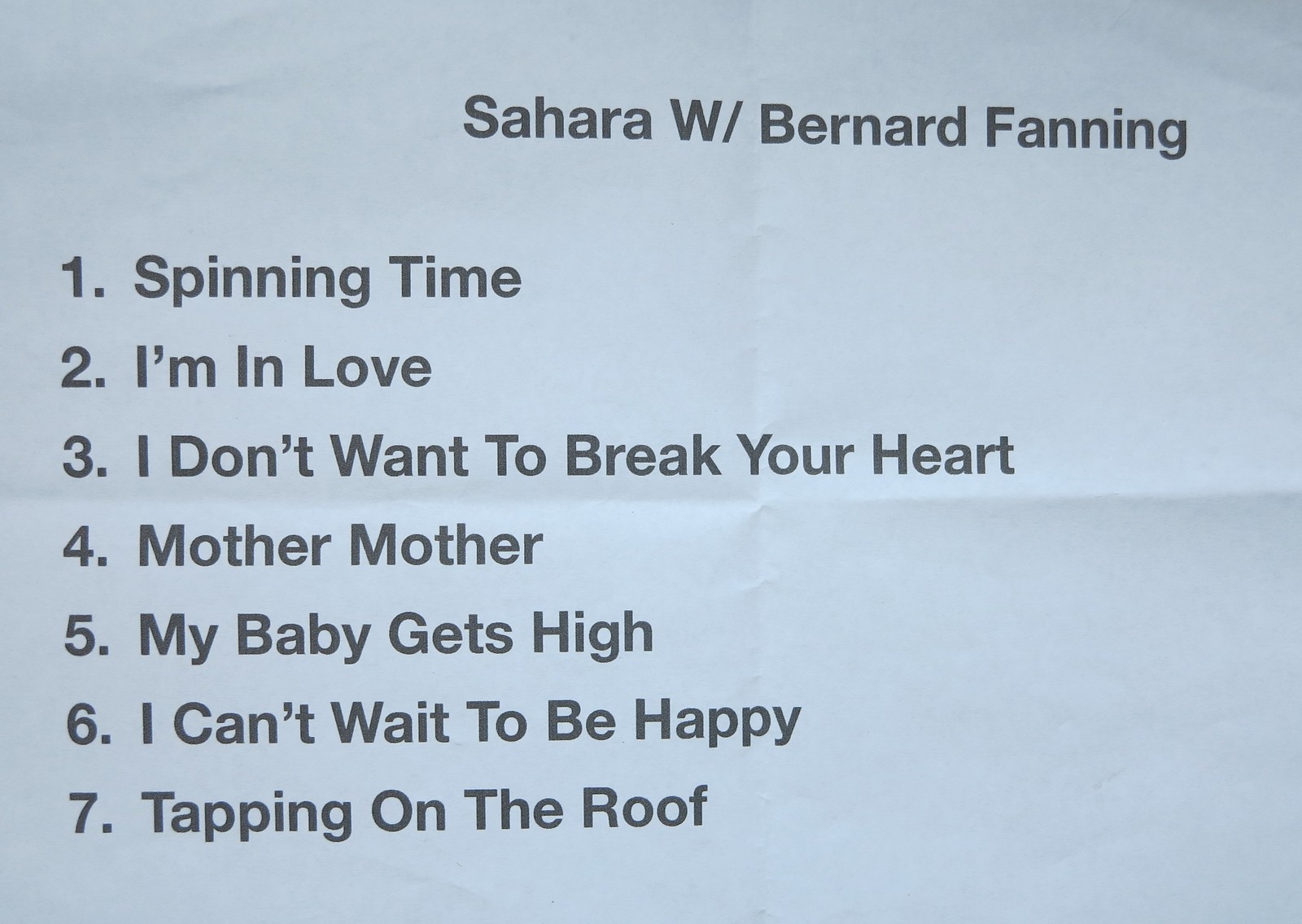The image displays a piece of paper with a slight grayish-blue hue and visible creases from being folded into quarters. The text, printed in black, lists a sequence of seven items, each accompanied by a number. Positioned in the top right corner, the title reads "Sahara w/ Bernard Fanning." The listed items on the left side include: 1. Spinning Time, 2. I'm in Love, 3. I Don't Want to Break Your Heart, 4. Mother Mother, 5. My Baby Gets High, 6. I Can't Wait to be Happy, and 7. Tapping on the Roof.